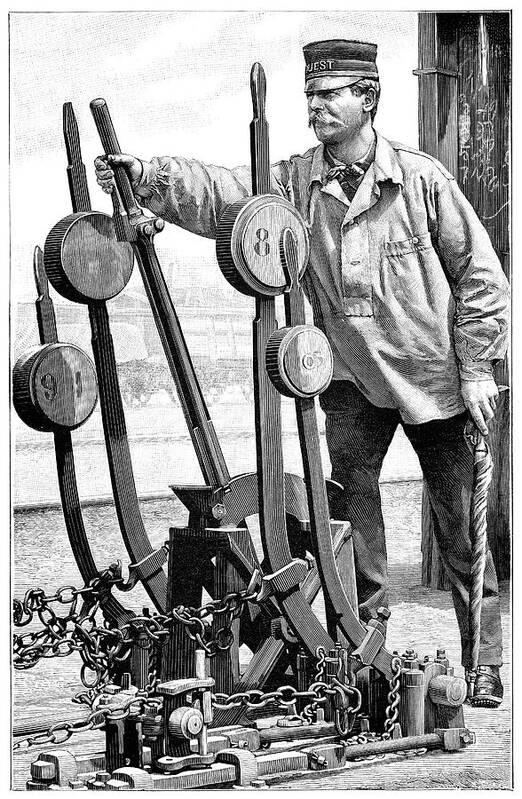This image is a highly detailed black and white drawing, resembling a 19th-century print, depicting a white man with a mustache. He is wearing a hat inscribed with the word "guest," which resembles a conductor's hat, and a loose-fitting button-down shirt. The man is centrally positioned in the image, standing at a set of six levers, and is engaged in pulling one of them with his right hand. This lever bears the numbers "8-5-9-1" and has chains at its base. In his left hand, he holds a pointed stick or cane. The background, appearing slightly foggy, features a faint depiction of a horse and buggy on a street, suggesting a historical setting. Additional elements include a wall with indistinct squiggles, contrasting the otherwise clear foreground. The overall composition and placement of elements emphasize the antiquated and industrial nature of the scene.